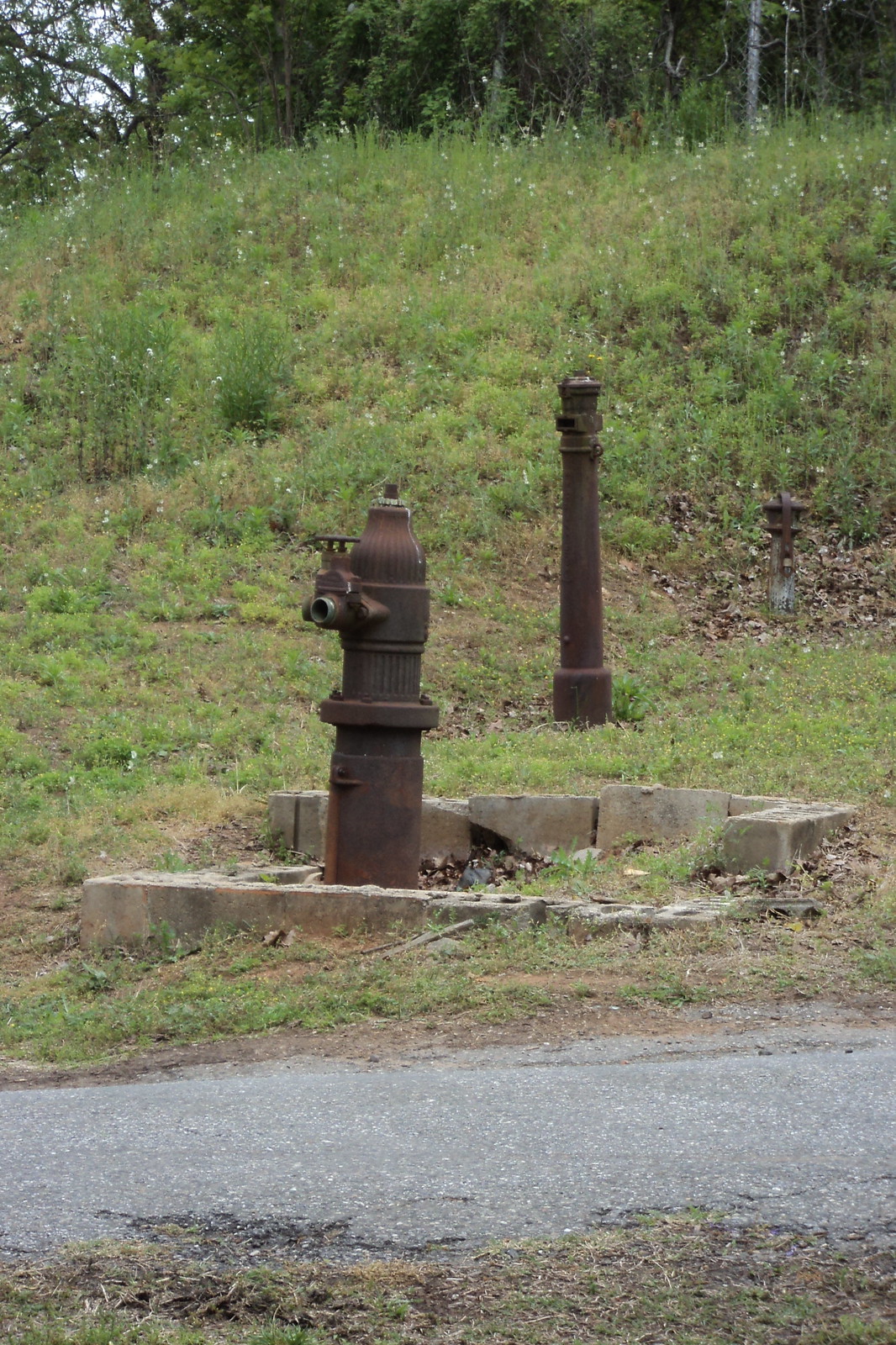The photograph captures an outdoor scene during the day, likely in the spring or summer months, or possibly in a tropical area, characterized by lush, green trees and shrubs with tall grass in the background. At the forefront, there are two cylindrical, tarnished brown structures resembling old water pumps or fire hydrants. The one positioned more forward is drizzling water and features a couple of turnable knobs. It is surrounded by cracked and disarrayed concrete blocks, indicating its age. Behind it, another similar cylindrical structure stands. Further in the background, partially obscured by the grass and trees, is a statue with a deer head, displaying a light gray color. A small pathway or road can be seen at the bottom of the image.